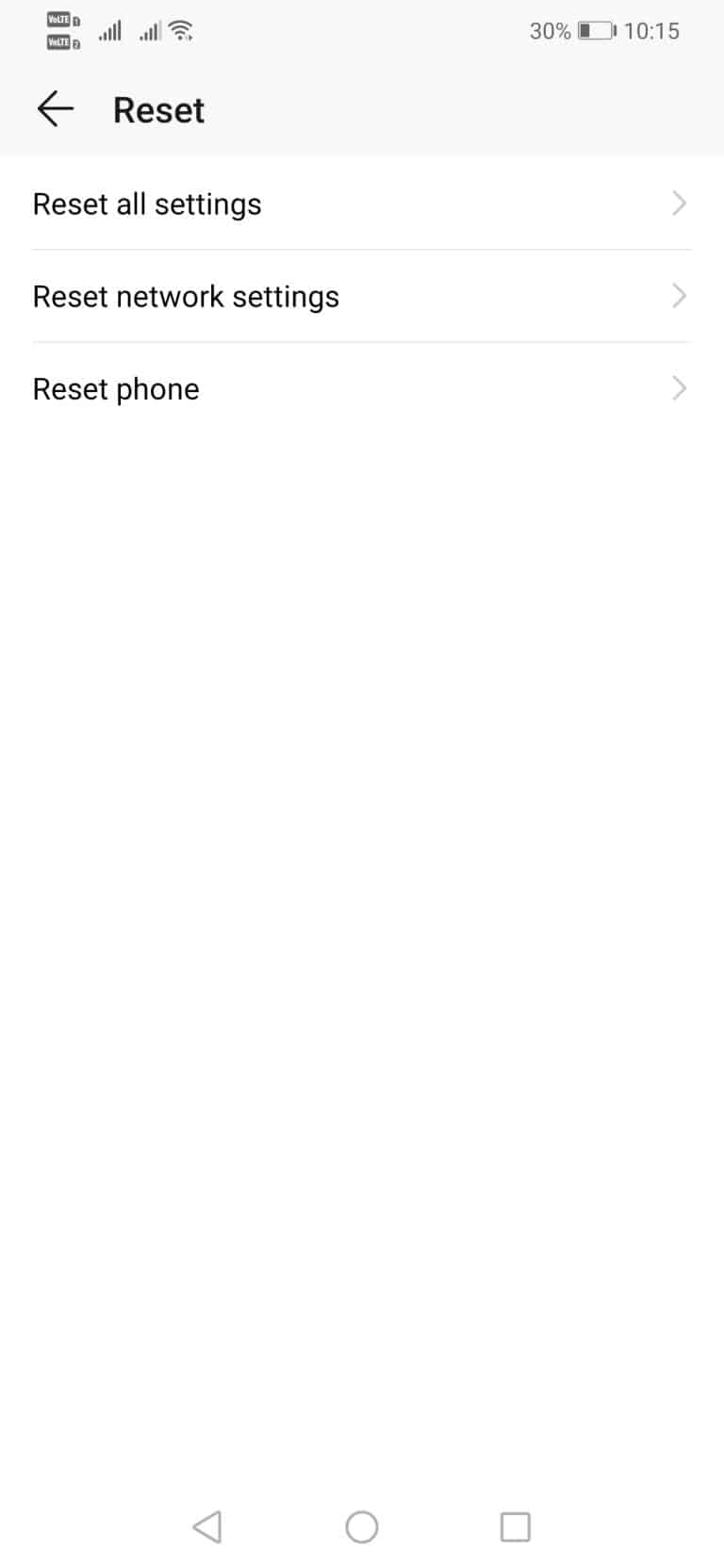The image depicts the screen of a smartphone displaying a "Reset" settings page. Although the smartphone itself isn't visible, it's clear from the interface elements. In the upper left corner, the time reads 10:15, with a battery icon showing 30% charge to its left. Dominating the image, the word "Reset" appears in the largest font, accompanied by a left-pointing arrow. Below, three reset options are listed vertically: "Reset All Settings," "Reset Network Settings," and "Reset Phone," each aligned to the left. To the right of each option is a right-pointing arrow. The entire background is white, with black text and a very light gray banner at the top.